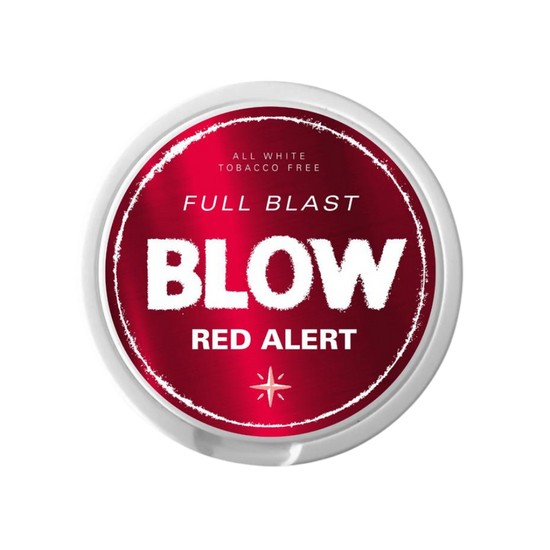The image is a top-down photograph of a circular container lid, likely for a jar or can. The lid has a distinct white border and is adorned with a dark red circular sticker at the center. This sticker features a series of stylized white texts. In the upper portion of the sticker, the text reads "ALL WHITE TOBACCO FREE" in capital letters. Below this, another line of text states "FULL BLAST," leading to the most prominent and bolded text "BLOW" in the center of the sticker. Directly beneath "BLOW," the words "RED ALERT" are displayed. Completing the design, there is a four-pointed star-like symbol at the bottom. The text "BLOW" appears to have a powdery texture, enhancing its visual impact.